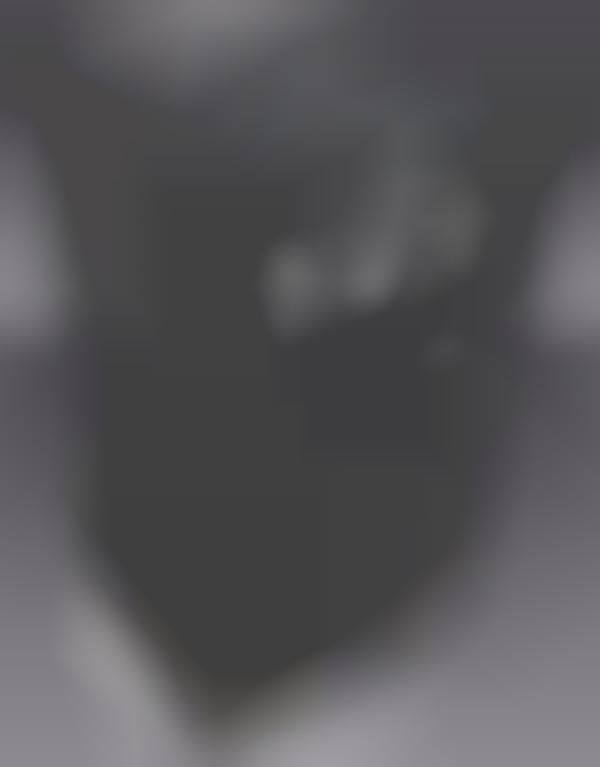This image is an extremely blurry satellite photograph taken from above, dominated by dense clouds that leave the edges white and gray. The majority of the image remains unfocused, with a large, indistinct dark mass in the middle that stretches downward, narrowing to a point past the halfway mark. Lighter gray and white areas appear scattered, especially towards the top right, resembling fragmented circles. The center, where the clouds thin slightly, reveals foggy flatlands with several indistinct structures, including a darker building towards the center and a lighter one towards the top left of this opening. Overall, the photo lacks clarity, making detailed identification of the terrain and structures difficult.